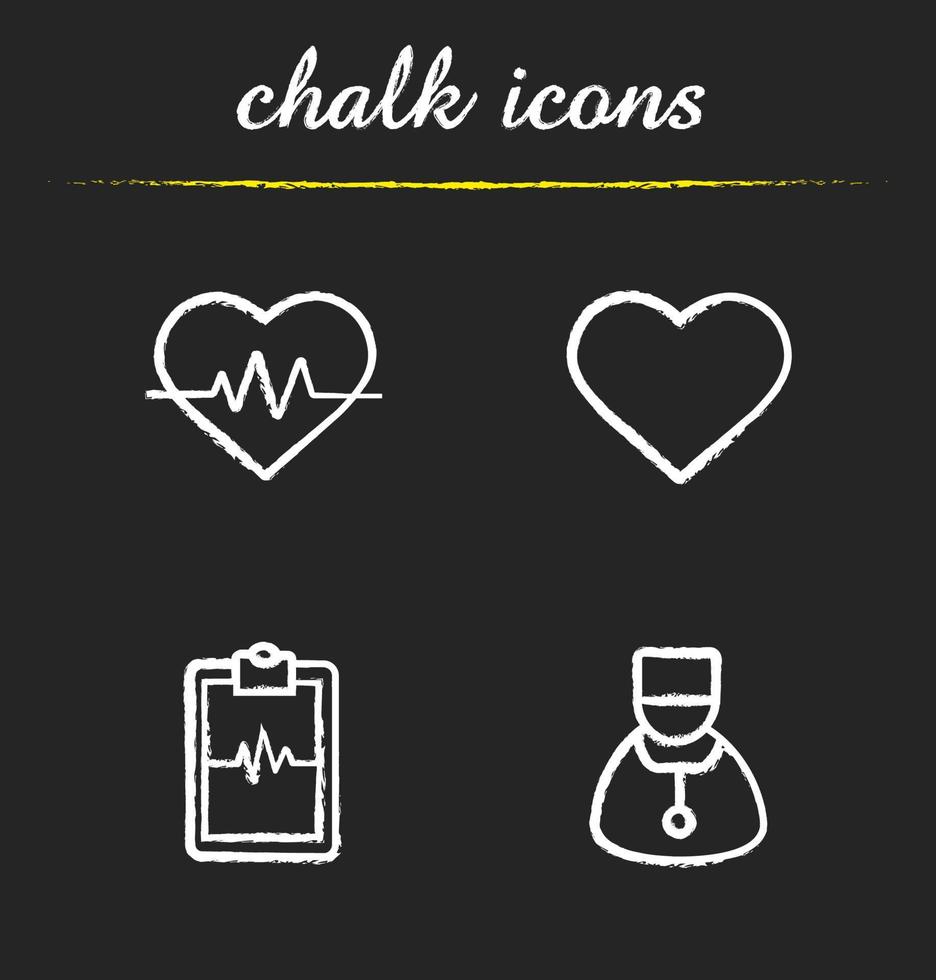The image is a black square with white, cursive text at the top that reads "chalk icons" in lowercase letters. Below this text is a bright, hand-drawn yellow line that appears slightly uneven, as if done with a pencil. The image features four white chalk-drawn icons arranged in two rows. In the first row, from left to right, there is a heart with an EKG line running through it and a standard heart with no lines. In the second row, on the left, there is a rectangular monitor displaying the same EKG line, and on the right, there is a coarse depiction of a medical figure, likely a nurse, wearing a hat and a stethoscope around their neck. The image utilizes only three colors: black, white, and yellow.